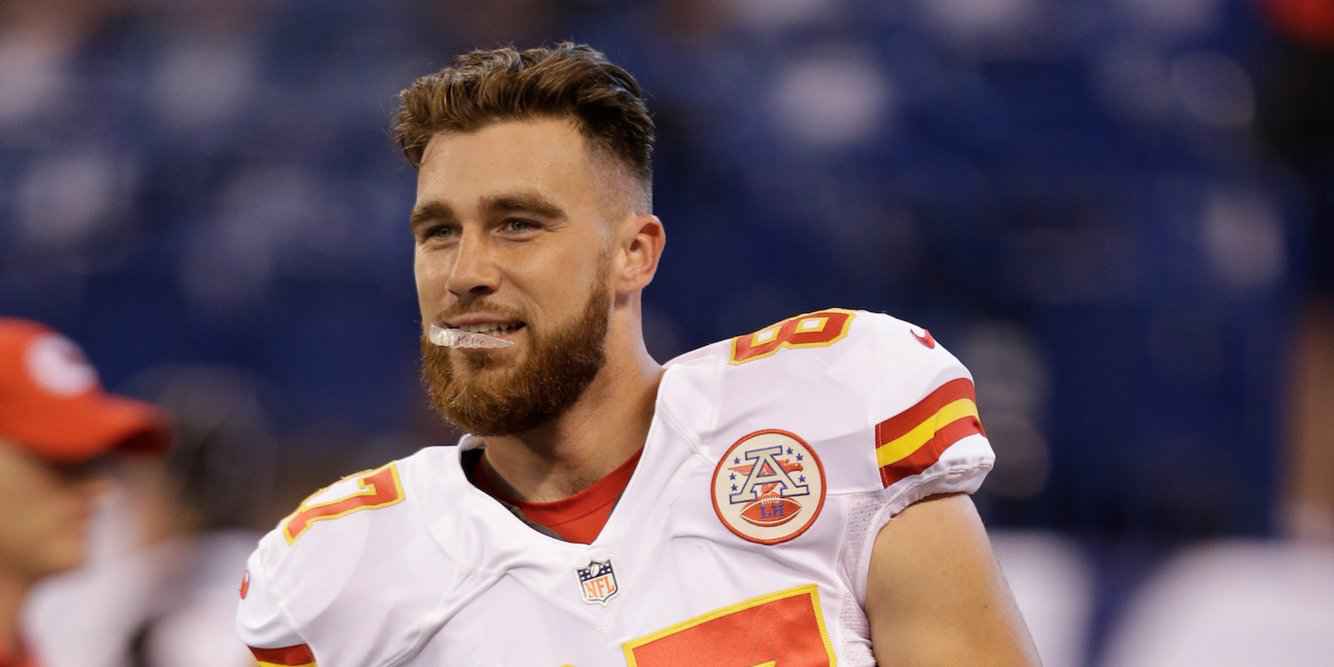This photograph captures NFL player Travis Kelsey, currently the boyfriend of Taylor Swift, in full uniform for a football game. Kelsey is dressed in the classic Kansas City Chiefs jersey, prominently featuring a white V with an A inside a white circle and a football beneath it on his chest. His uniform is primarily red and yellow with his number 87 displayed—broken up into 7 on his left shoulder and 8 on his right. Kelsey’s short, brushed-back brown hair and full medium-brown beard frame his face, where he holds a clear or white mouth guard between his teeth, obscuring part of his facial expression. His eyes, potentially a dark blue or green, look off to the left while his head is slightly turned in that direction. The background is heavily blurred, showing hints of blue seating in the stands and possibly a coach in a red baseball cap on the bottom left, along with other indistinct figures.